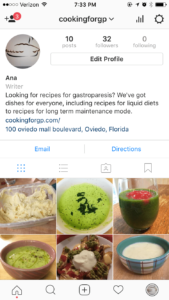The image is a screenshot taken from a cell phone, displaying an informational layout on a white background adorned with black text. The screenshot is vertically oriented and intuitively organized.

At the top of the display, the status bar reveals the Verizon network along with the current time situated in the center. Directly beneath the time, a heading reads "Cooking for GP." On the upper left, there is a circular icon resembling a sphere with interwoven white and black lines, indicative of a logo or emblem.

Following this, the text identifies the author as "Anna, Writer" and introduces the subject matter: "Looking for recipes for gastroparesis." The main body of text elaborates on the variety of recipes available, catering to everyone with options that range from liquid diets to long-term maintenance meals.

Highlighted in blue text is the website URL, "cookingforGP.com," along with the address "100 Aviato Mall Boulevard, Aviato, Florida." Beneath this, clickable blue text options "Email" and "Directions" provide interactive elements likely aimed at further engagement.

At the bottom of the screenshot, there are six images of food items. The images are arranged in two rows, each containing three pictures:
1. On the top left, there is a container of what looks like potato salad.
2. The top middle image shows a white bowl filled with green soup.
3. The top right image features a green container with a red liquid inside.
4. On the bottom left, there is a brown bowl filled with green soup or mush.
5. The bottom middle image displays a white plate with a mix of green and red food items, topped with a dollop of something white in the center.
6. The bottom right image shows a blue plaid-patterned bowl containing a white liquid.

This detailed caption meticulously outlines the visual and textual elements of the screenshot, providing a comprehensive understanding of the content and layout.